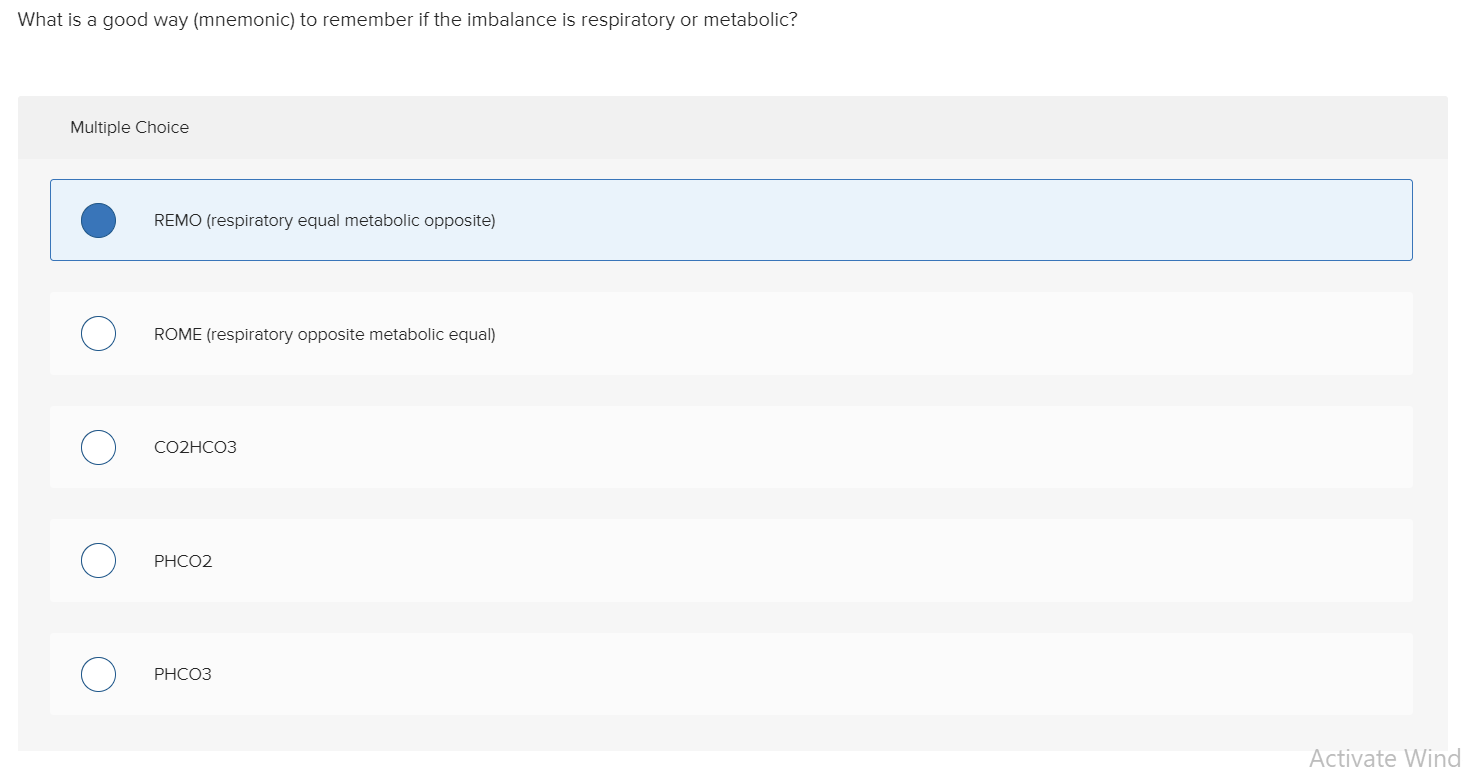The image is a screenshot of a minimalist questionnaire website with a white background. At the very top, there is a question displayed in bold text asking, "What is a good way (MNEMONIC) to remember if the imbalance is respiratory or metabolic?" Below the question, there are five multiple-choice options presented with radio buttons beside each one.

The first option has its radio button selected, and the text beside it reads "REMO" in capital letters, followed by "(Respiratory Equal, Metabolic Opposite)" in parentheses. The subsequent option is labeled "ROME" in capital letters, with "(Respiratory Opposite, Metabolic Equal)" in parentheses. The third option reads "CO2HCO3" in all caps. The fourth option, also in all caps, is "PHCO2." The final option is labeled "PHCO3" in all capital letters. Each of these choices suggests different mnemonic strategies for distinguishing between respiratory and metabolic imbalances.